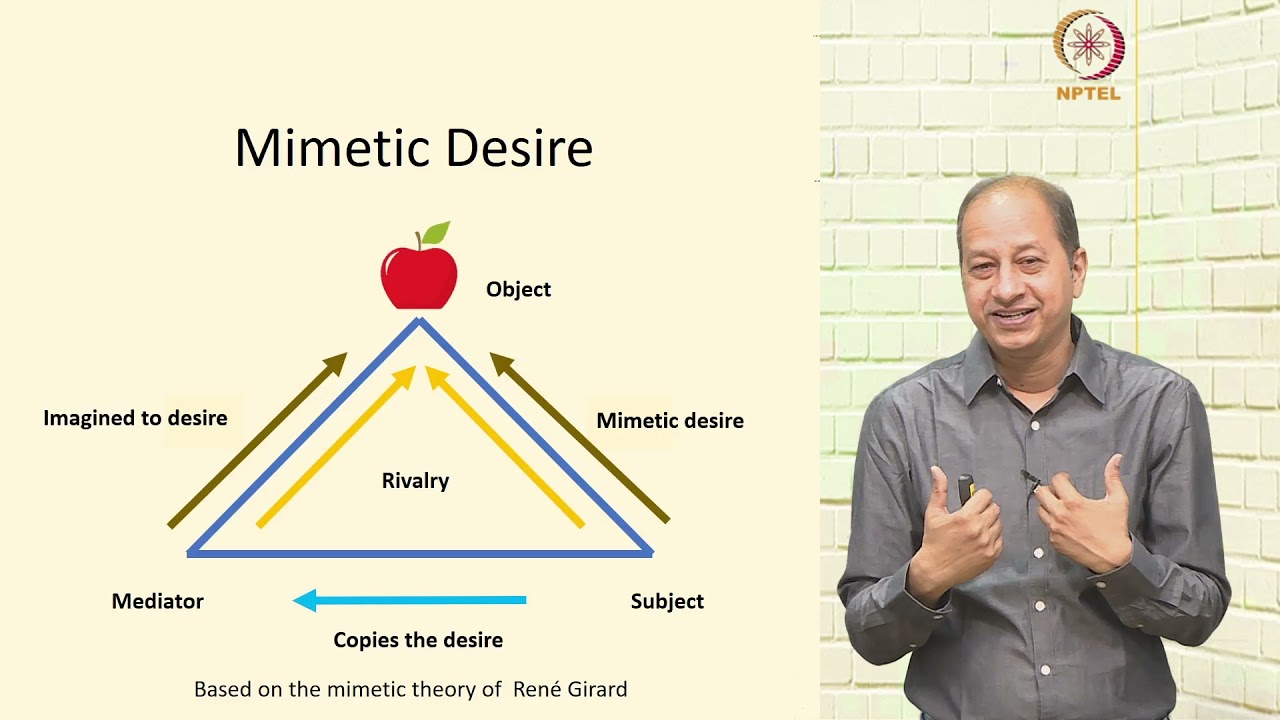In this detailed image, we observe a presentation slide likely captured from a video, where a man in a gray button-down shirt is explaining the concept of mimetic desire based on the theory of René Girard. The right-third of the image features this presenter, who appears to be of Southeast Asian descent, standing against an off-white brick background and gesturing with open palms. The NPTEL logo, resembling an atomic star within two crescents, is also visible at the top right.

The left two-thirds of the image contain a detailed infographic. At the top, the term "Mimetic Desire" is prominently displayed with an apple labeled "Object" beneath it. Surrounding the apple, a network of arrows and labels elucidates the relationships in mimetic theory. A blue triangle sits at the core with various arrows indicating interactions: yellow arrows inside the triangle point upward labeled "rivalry," brown arrows on the perimeter indicate "Imagined to Desire" on the left and "Mimetic Desire" on the right. A blue arrow at the base of the triangle, labeled "Copies the Desire," points to "Subject," while below the triangle, "Mediator" and "Subject" are positioned on either side with respective labels. The entire diagram visualizes the dynamics of desire, with the core message that desires are copied, structured within the confines of René Girard's theory.

Overall, the image encapsulates a scholarly discussion on mimetic desire, effectively combining graphical representation and personal presentation to engage the audience.